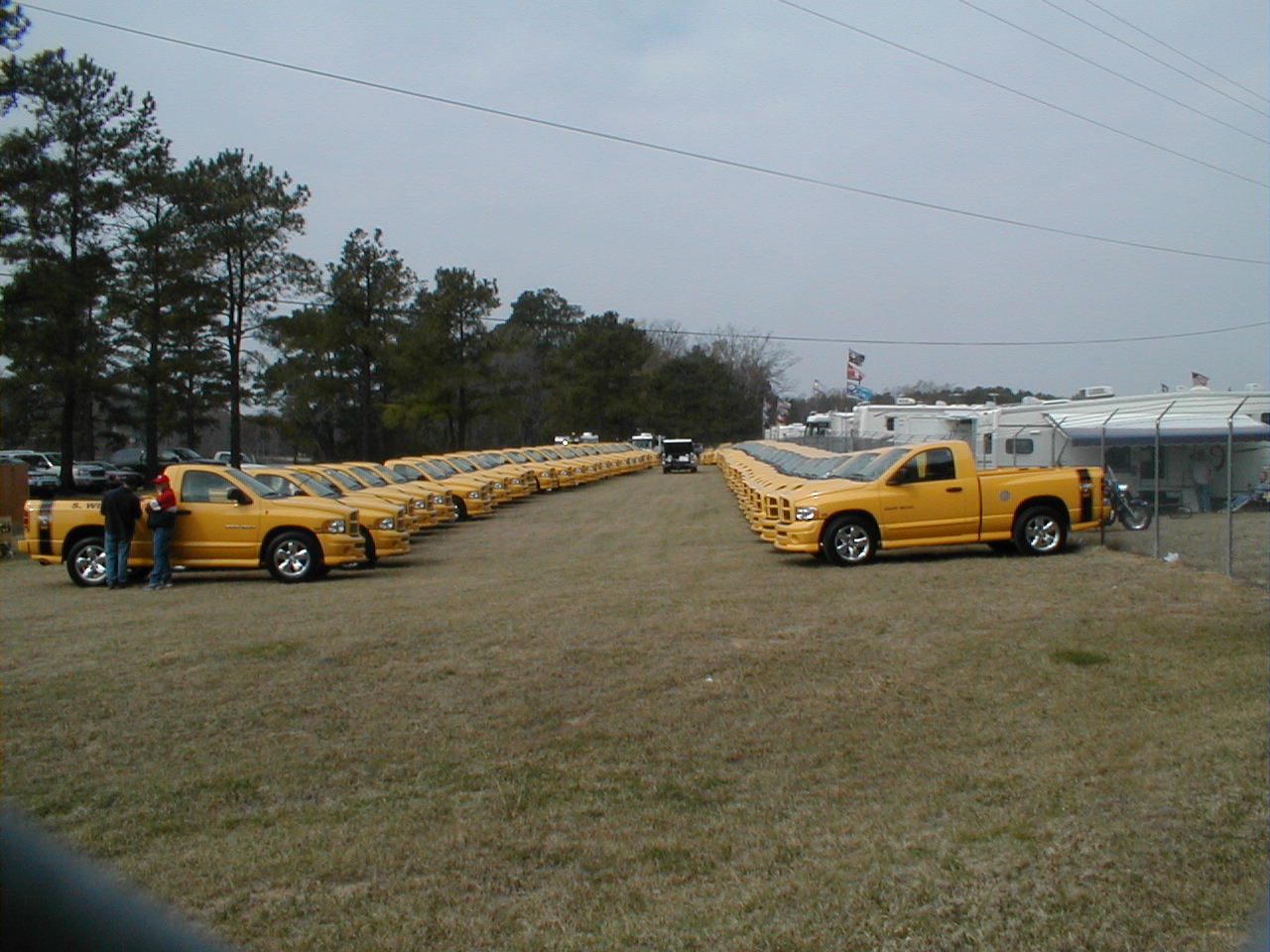This outdoor color photograph, taken during an overcast day, features two lines of identical yellow pickup trucks facing each other, with their bumpers almost meeting. The trucks, all two-door models with short beds and chrome wheels, form rows extending into the background. The space between the rows is approximately 25 feet wide and is filled with slightly browned, freshly mowed grass. In the foreground, the grass continues, while utility lines run horizontally across the upper portion of the image.

To the left behind the trucks, there is a line of tall, green trees, while on the right side, a chain-link fence is visible. Beyond the fence lies an RV park with several white RV trailers and a motorcycle. In the background, three flags of different colors—black, red, and blue—can be seen. Additionally, standing off to the left are two people; one of them is dressed in a red shirt and cap, and the other in a black shirt. Both individuals are wearing jeans.